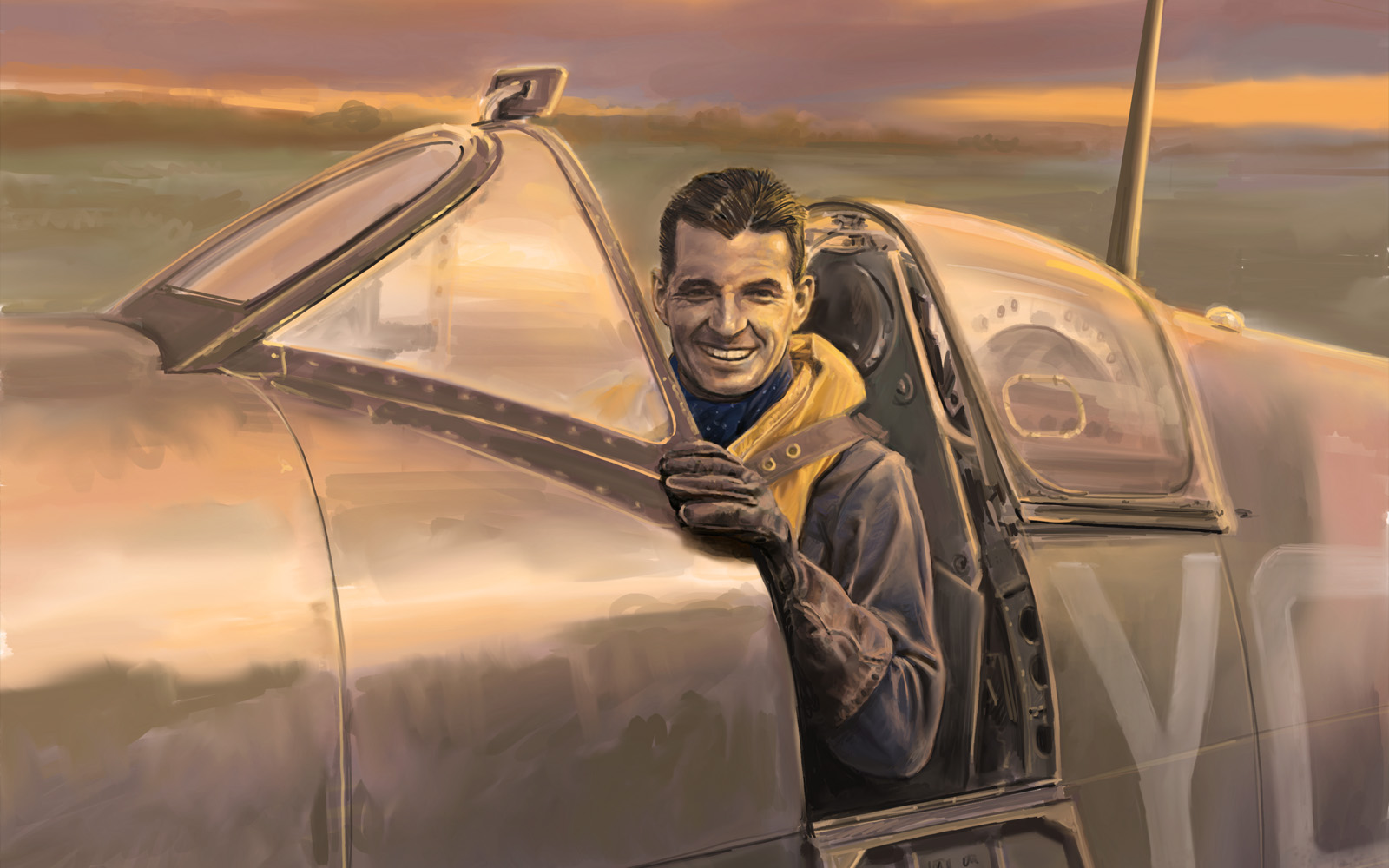In this detailed illustration, the viewer sees a man sitting on the outer portion of an older-style airplane, possibly a war plane, which is rendered in a muted, washed-out grey-brown color. The airplane's metallic surface has a color gradient, indicating its reflective nature, and bears the partial markings "Y" and another cut-off letter. The background is a serene sunset with pale pastel hues, orange clouds, and hints of green grass beneath a darkening sky. The man, who is in a seated position facing the viewer, smiles warmly. He is adorned in a yellow vest, brown leather gloves, a long-sleeved leather jacket, a yellow scarf, and a satchel, with short hair that complements his cheerful demeanor. The overall piece has a watercolor-like softness, blending hues seamlessly across the image, which is longer in width than in height.